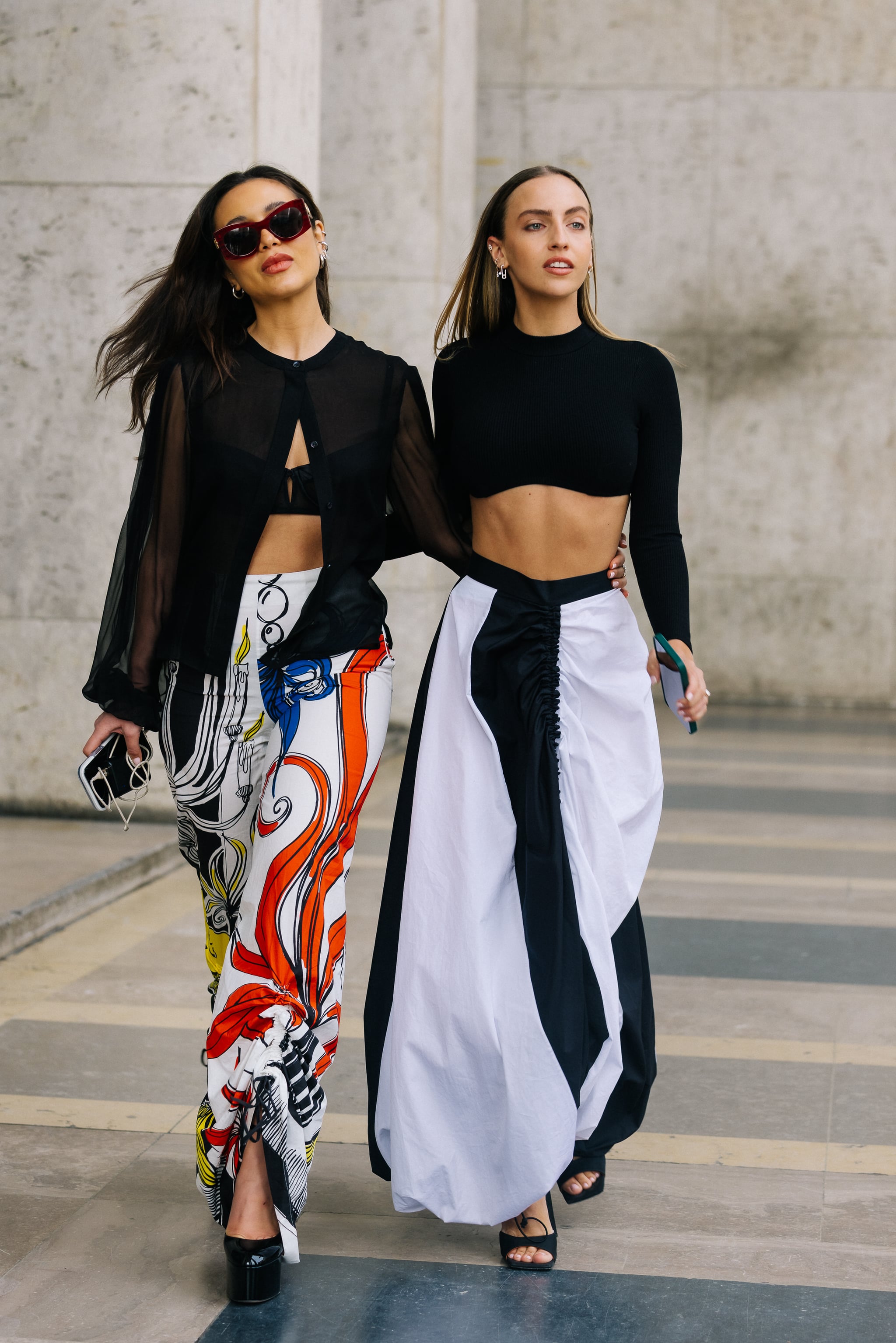In this image, two young women are walking side-by-side on a shiny concrete or cement surface that features yellow and bluish-green lines. They are in a crosswalk or sidewalk area with a white-gray background punctuated by black or gray spots. The woman on the left has long dark hair and is wearing red-rimmed sunglasses. She is dressed in a black split top that reveals her midsection and colorful pants with designs in blue, red, yellow, and white. She is holding a black and white cell phone and a power bank in her right hand, and wears black shoes. The woman on the right has a slightly lighter hair color and is dressed in a black long-sleeve crop top paired with a white and black skirt. She is also wearing black sandals. The two women have their arms wrapped around each other's backs as they walk together.